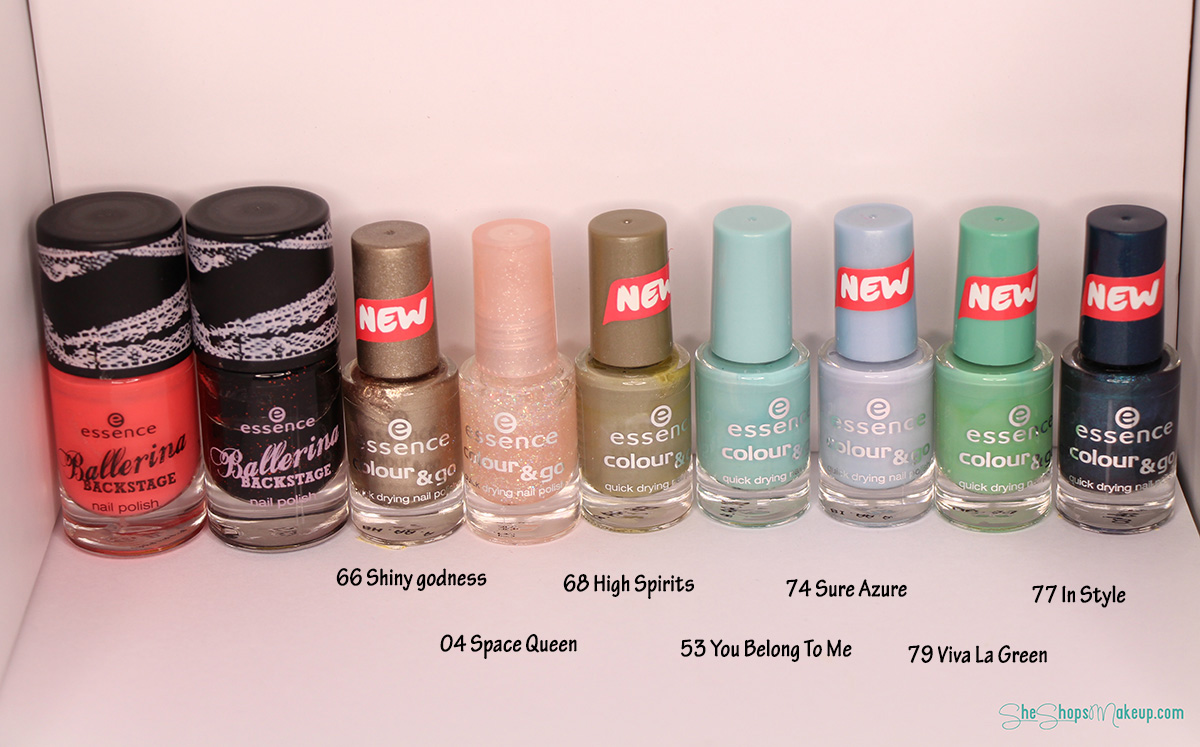The photograph showcases a neatly arranged display of nail polish bottles, set against a white cardboard backdrop. The image features a total of nine little bottles, with varying colors and finishes, laid out from left to right. Two larger, unlabeled bottles on the far left are notable for their distinct sizes, with one appearing orange and the other black. The remaining seven bottles are smaller with long, thin caps and are labeled with both names and numbers: 66 Shiny Goddess, 04 Space Queen, 68 High Spirits, 53 You Belong to Me, 74 Sure Azure, 79 Viva La Green, and 77 InStyle. These labels do not all indicate the color explicitly, except for 'Sure Azure,' and 'Viva La Green.' The bottles exhibit a diverse palette including hues of red, pink, blue, green, and purple, with some featuring shiny textures. Beneath each bottle, different codes and names are displayed. At the lower right corner, a URL reads "seashopsmakeup.com", identifying the source or brand.